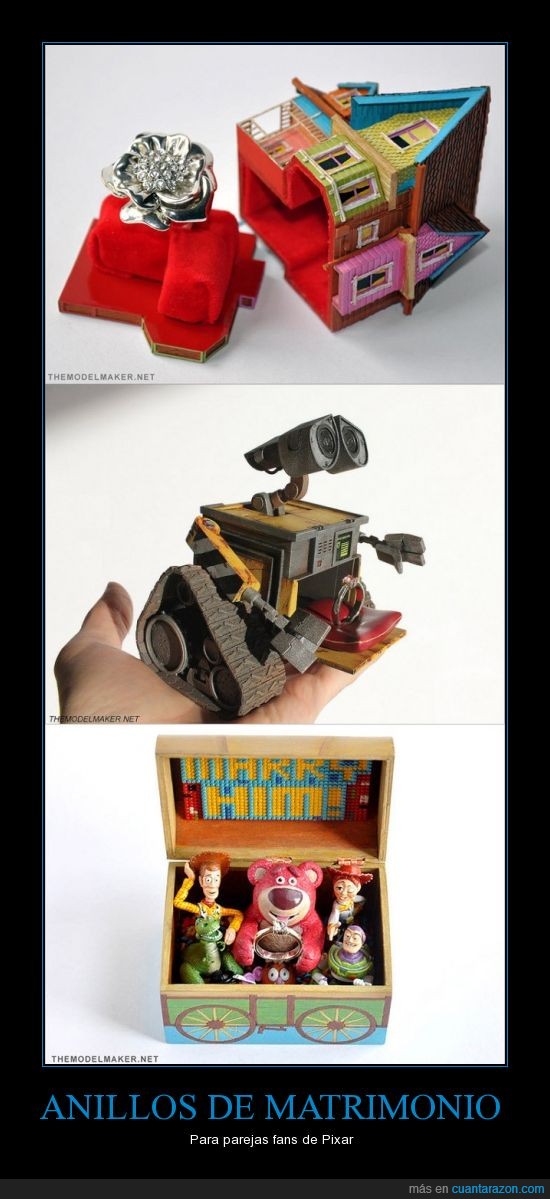This image depicts a promotional poster titled "Anillos de Matrimonio para Parejas Bands de Pixar," featuring three detailed and vibrant images of children's toys re-purposed as unique ring boxes.

In the top image, a colorful dollhouse is flipped over on its side, revealing a red base with a silver metal piece, creatively doubling as a ring holder. 

The middle image showcases a hand holding a toy depiction of WALL-E, the beloved Disney character from the Pixar movie. The toy has a hidden compartment in its torso under its eyes, perfect for concealing a ring. 

The bottom image displays a wooden toy chest adorned with sketched bicycle wheels on its front. Inside the chest are Toy Story characters: Woody, the cowgirl Jessie, Buzz Lightyear, and Lotso the pink bear. The top of the box features text spelled out in Lego-like blocks, reading "Marry Him."

This inventive amalgamation of popular children's toys and romantic elements symbolizes the joy and nostalgia of Pixar films while presenting a whimsical approach to proposals.